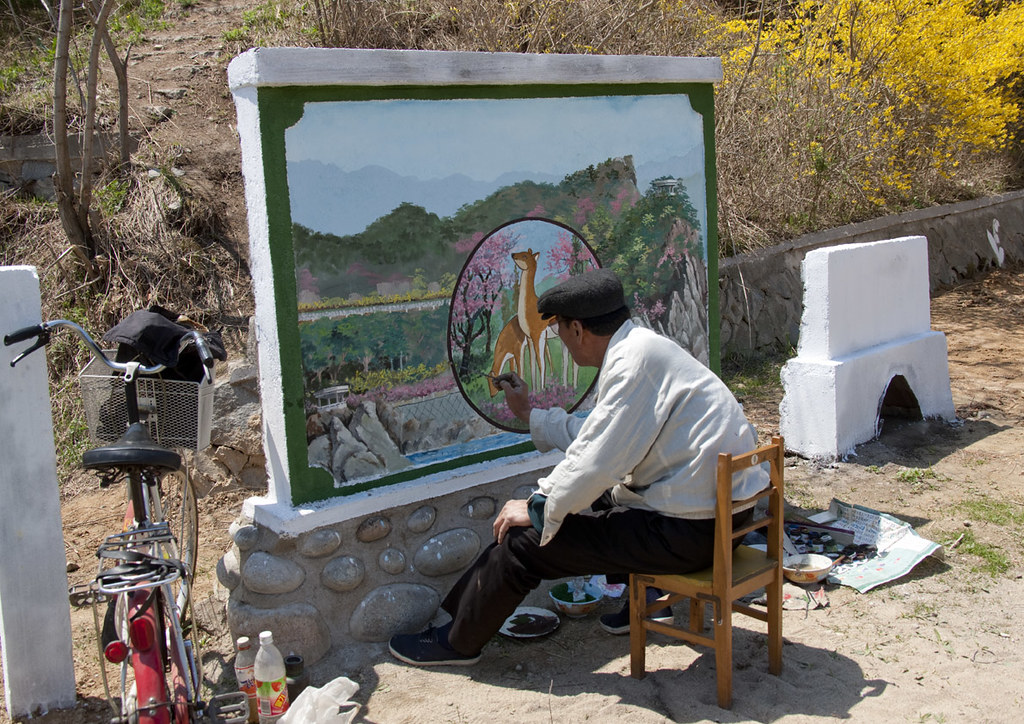In this horizontal color photograph, a man is seated on a small wooden chair outdoors, immersed in painting a mural on a concrete segment that rests on a stone base. The mural, approximately the size of a dining table, depicts a scenic landscape of trees and mountains, with a circular inset featuring two deer—one grazing and the other standing alert. The artist, dressed in a hat, long shirt, and pants, holds a paintbrush as he works. Surrounding him are various painting supplies, including bowls filled with paint and a paper filled with paintbrushes. Nearby, a red bicycle with a basket holding a bag is parked, alongside some plastic bottles. The setting is a natural environment with barren dirt, bushes—some adorned with yellow flowers and others lifeless—and a trail that meanders into the woods in the background.